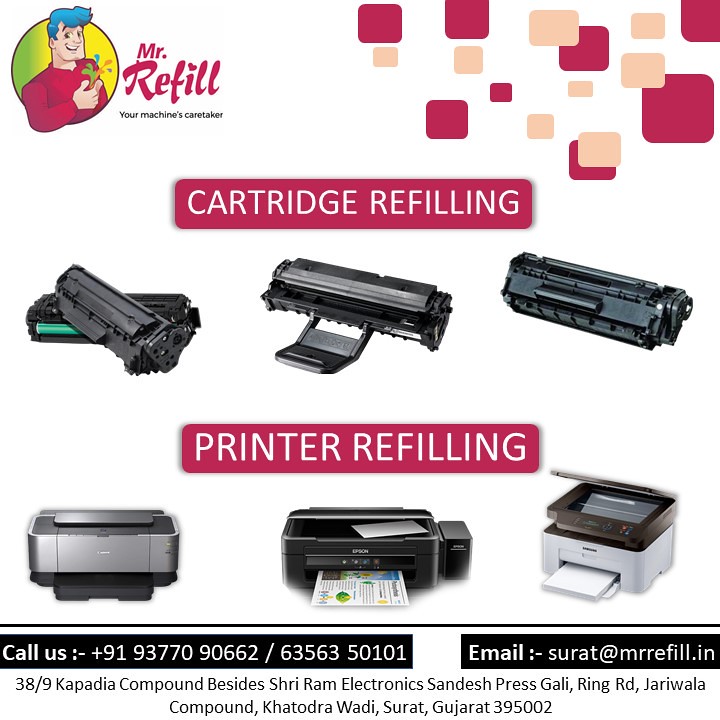This advertisement poster features a prominent and neatly organized layout against a white background, promoting cartridge and printer refilling services. At the top left corner, there is a circular logo of a cartoonish character named Mr. Refill, a beefy figure wearing a red shirt and sporting blue hair, alongside the tagline "Your Machine's Caretaker." Directly to the right of this logo, bold text spells out "Cartridge Refilling" in white letters against a pinkish-red background, accompanied by images of three cartridge components. Below, the phrase "Printer Refilling" follows the same design scheme, displaying three variously shaped and sized printers. The bottom section of the ad provides detailed contact information, including a phone number, an email address, and an area code of 395002, complemented by concise directions to their location. This well-balanced and visually appealing ad is suitable for display in magazines or as a standalone poster.